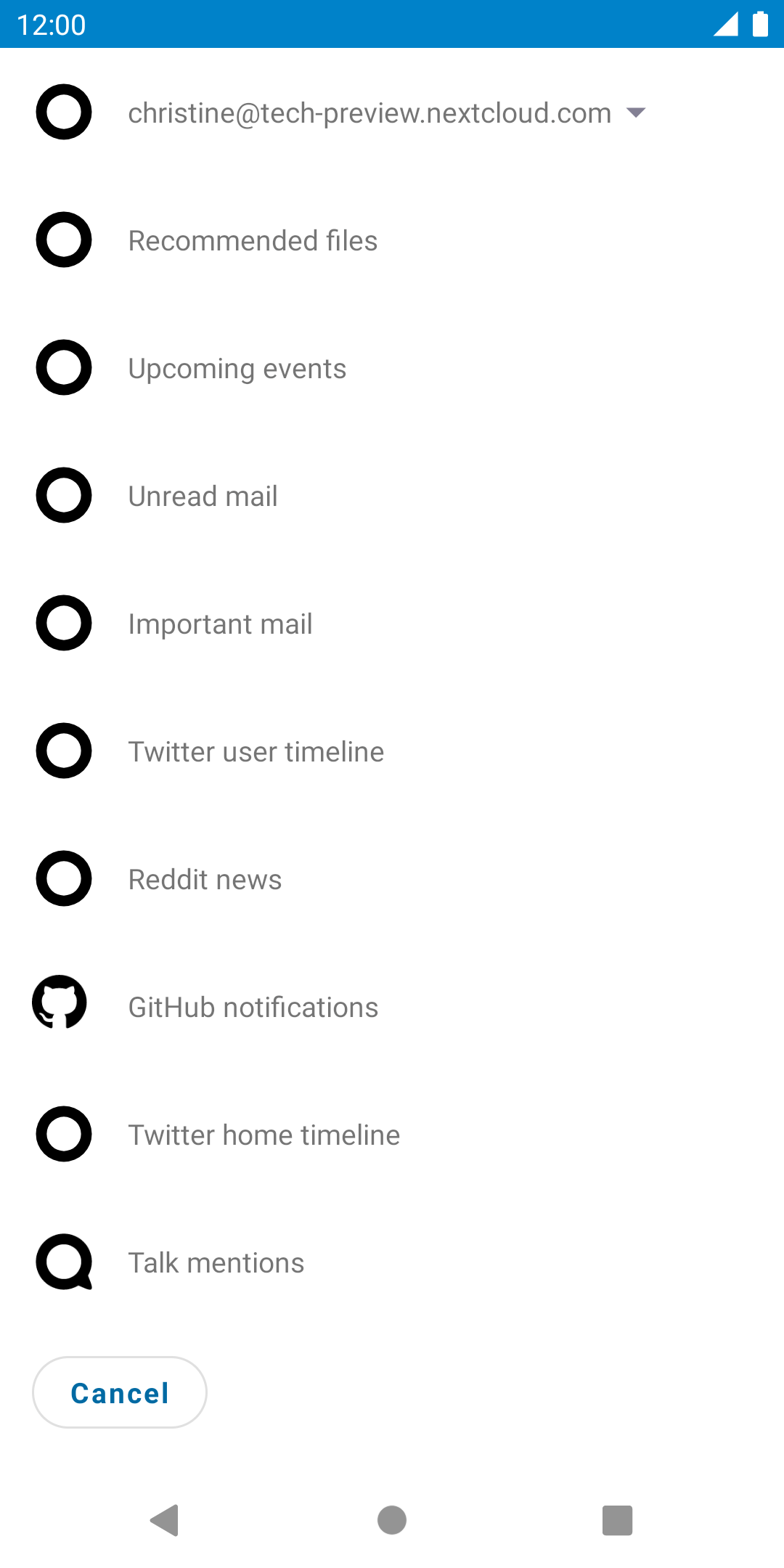The image appears to be a screenshot from a smartphone. At the very top, there's a blue bar displaying the time, which is 12:00. On the left side of the bar, the time is clearly visible, while the top right corner shows the signal strength and battery level, both of which are completely full and displayed in white.

Below this blue bar is a series of options, each accompanied by a circle to their left. Most of these circles are outlined in black, while several contain small icons. The first option reads "Christine at tech-preview.nextcloud.com" and features a down arrow next to it. The subsequent options are organized as follows:

1. Recommended Files
2. Upcoming Events
3. Unread Mail
4. Important Mail
5. Twitter User Timeline
6. Reddit News
7. GitHub Notifications
8. Twitter Home Timeline
9. Talk Mentions

At the bottom of the list, there is a button outlined in gray with blue text that reads "Cancel." Lastly, at the very bottom of the image, there are three navigation icons aligned horizontally: an arrow pointing to the left, a circle, and a square, all rendered in gray.